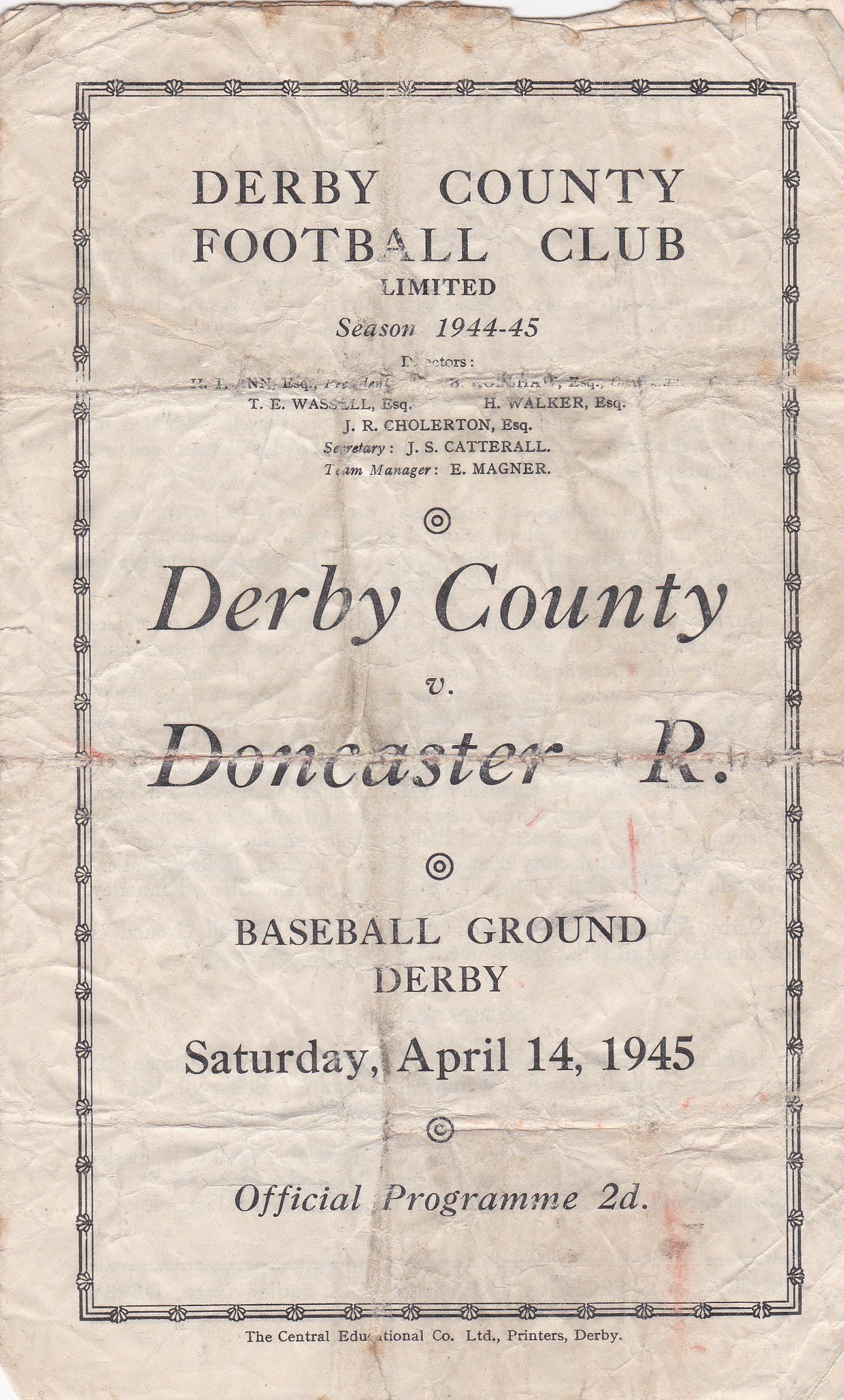The image shows a deeply wrinkled and worn-out piece of paper, indicating its age and extensive handling over time. The paper is tattered around the edges with deep crease lines from being folded and unfolded multiple times. It is predominantly white with black lettering, displaying the heading "Derby County Football Club Limited, Season 1944-1945" at the top. In larger, bold letters at the center, it reads "Derby County vs. Doncaster R." Beneath this, it states the location and date of the event: "Baseball Ground, Derby, Saturday, April 14, 1945." At the bottom, the words "Official Program, 2D" are visible. The lettering is framed by a decorative border featuring small pictures of shells, adding a unique touch to the design. This flyer is an official program from 1945, promoting a soccer match between Derby County and Doncaster R., held in Baseball Ground, Derby.